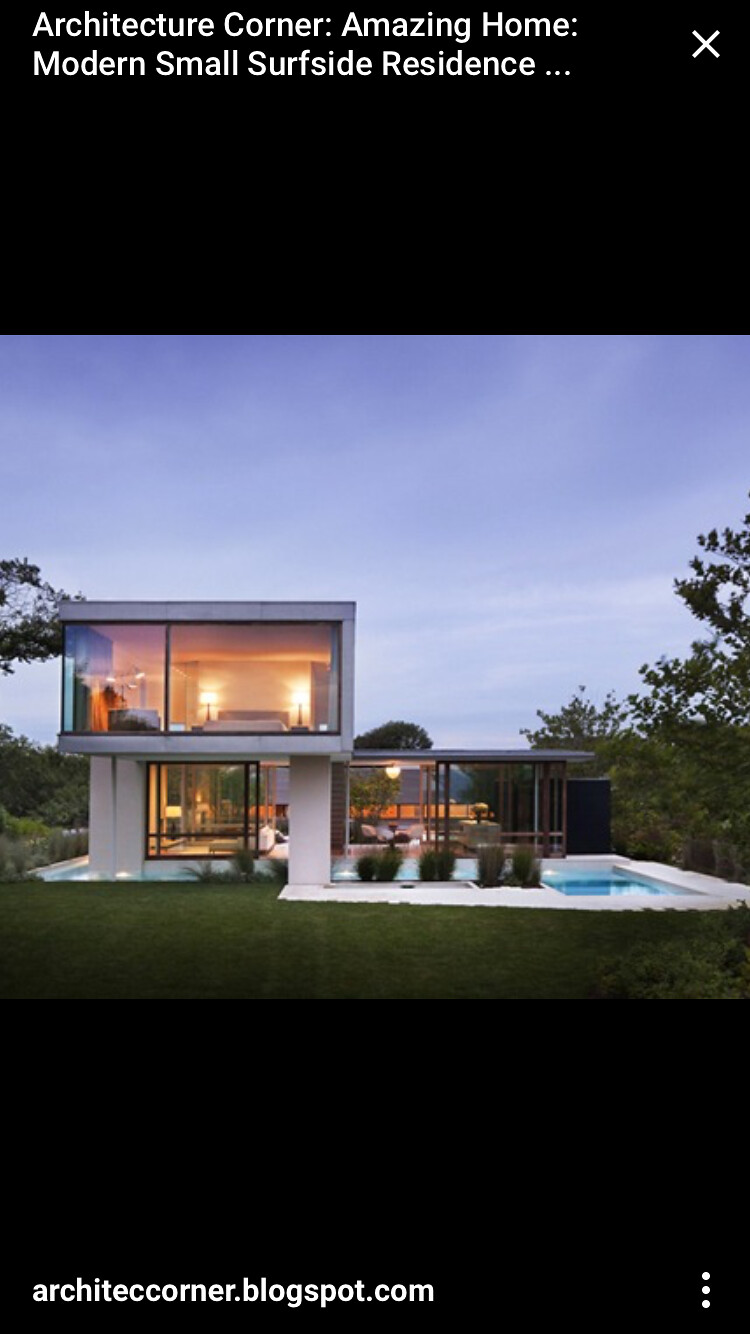The image showcases a stunning, modern two-story residence in the early evening, captured in a computer-generated graphic that appears to be from a blog or social media post. At the top of the black-bordered screenshot, white text reads "Architecture Corner: Amazing Home, Modern Small Surfside Residence." The black border at the bottom displays "architectcorner.blogspot.com" in white letters. The main subject is a sleek modular house with expansive floor-to-ceiling glass windows, providing a clear view into a glass-encased living room on the first floor and a glass-walled bedroom on the second floor. The bed in the bedroom faces outward, flanked by two lamps. Surrounding the house is a neatly manicured green lawn, and in the background, trees and a bright blue sky with a few clouds enhance the serene setting. To the right of the house, a striking blue in-ground pool extends across the property, suggesting a space designed for recreation and relaxation.